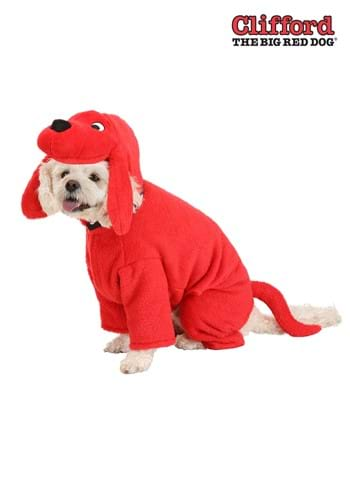This professionally photographed image features a small, light whitish-brown dog, possibly a schnauzer, dressed in a detailed and vibrant Clifford the Big Red Dog costume. The dog, with its dark black beady eyes, brown nose, and its pink tongue playfully sticking out, sits against a plain white background. The costume envelops the majority of the dog’s body, with a red hoodie-like design that includes Clifford’s iconic facial features—black and white eyes, a big black nose—and floppy red ears that drape down the sides of the dog’s head. Additionally, the costume has a red tail that aligns with the dog's own tail. In the upper right corner, in bold lettering, it reads "Clifford the Big Red Dog" with "Clifford" in red and "the Big Red Dog" in black, and includes the franchise's official logo. The overall composition, void of other text or context, suggests this image is an advertisement potentially associated with the Clifford franchise, showcasing either the costume or related merchandise.